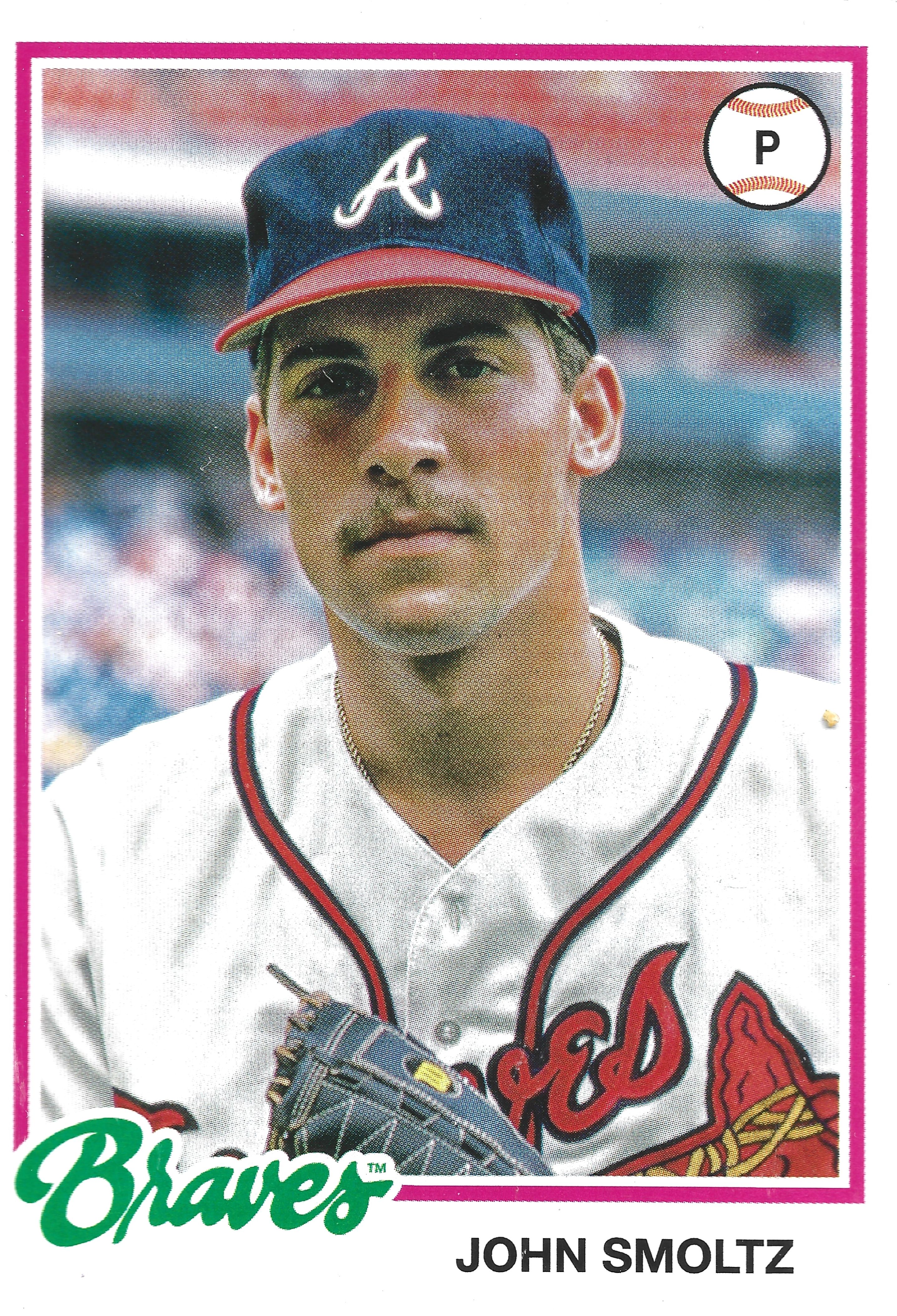This is a detailed and descriptive caption for the image:

The image features a baseball card from the 1990s showcasing John Smoltz of the Atlanta Braves. The card has a distinct pink border with an additional white inner border. John Smoltz is seen up close, wearing a blue cap with a red brim, adorned with a white "A" on the front. His white jersey features "Braves" written in red cursive with a tomahawk beneath the name, though part of the text is obscured by his brown baseball glove with tan stitching. Smoltz sports a silver chain and a mustache. In the top right corner of the card, there is a white baseball with red stitching and a black "P" on it. The background of the image is blurred, depicting the stadium and audience. The name "John Smoltz" is clearly printed in black letters at the bottom right corner of the card. The team name, "Braves," is also repeated in green type at the bottom left corner of the image.